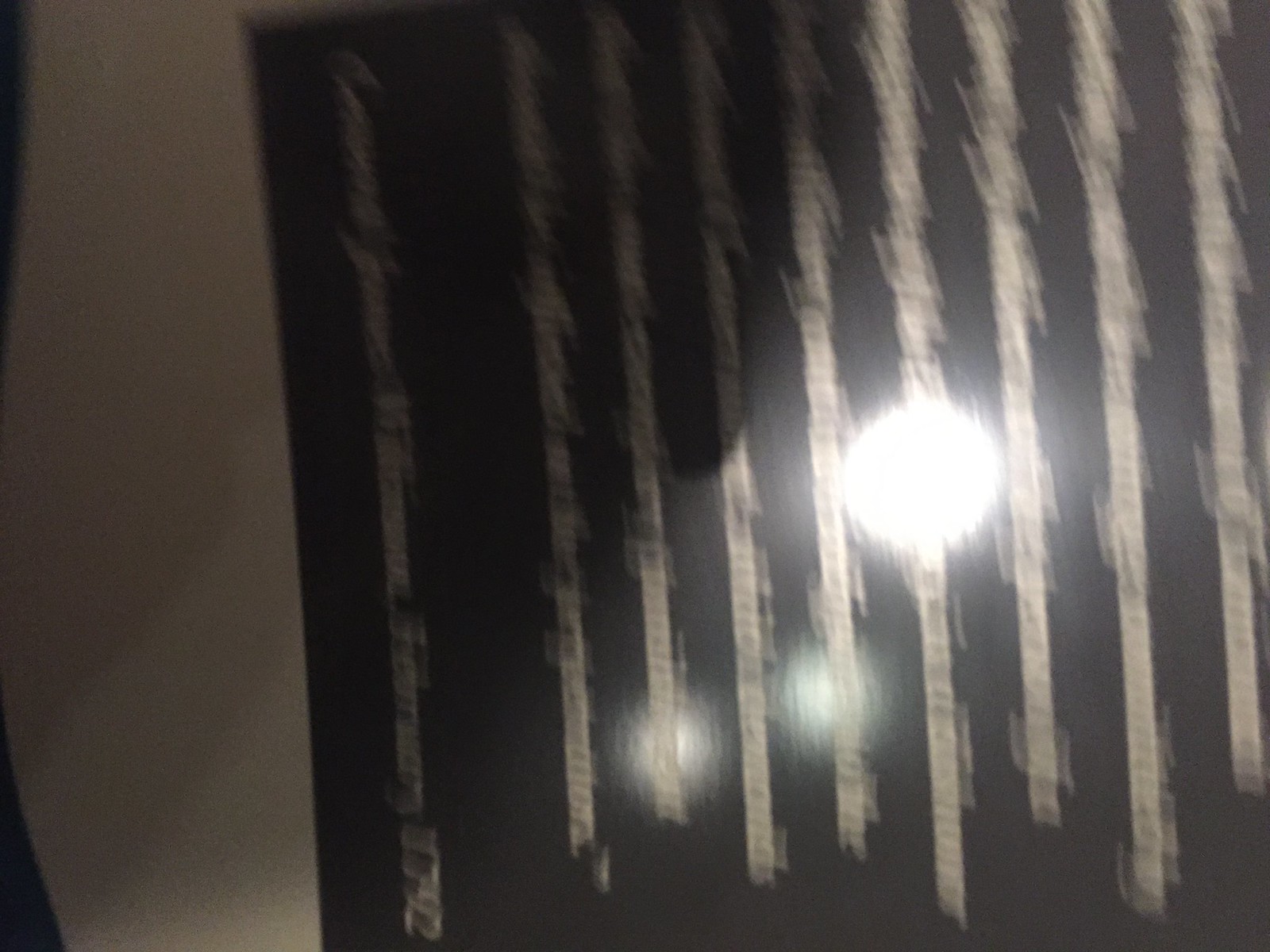The image features a dark background, possibly black or dark brown, with a glossy texture. Taken at night with a flash, the photo is extremely blurry and has been rotated clockwise. Dominating the left third is a large, bright white orb of light, likely a result of the camera flash, with two smaller, less bright orbs below it. The background displays vertical lines of white or silvery writing, creating a stark contrast against the dark backdrop. These lines are presumed to convey a name and a date, with "February 1792" and the potential last name "Williamson" discernible amidst the blur. The text appears on a board or plaque, likely from a museum setting, although the specifics remain obscured due to the image's poor quality.